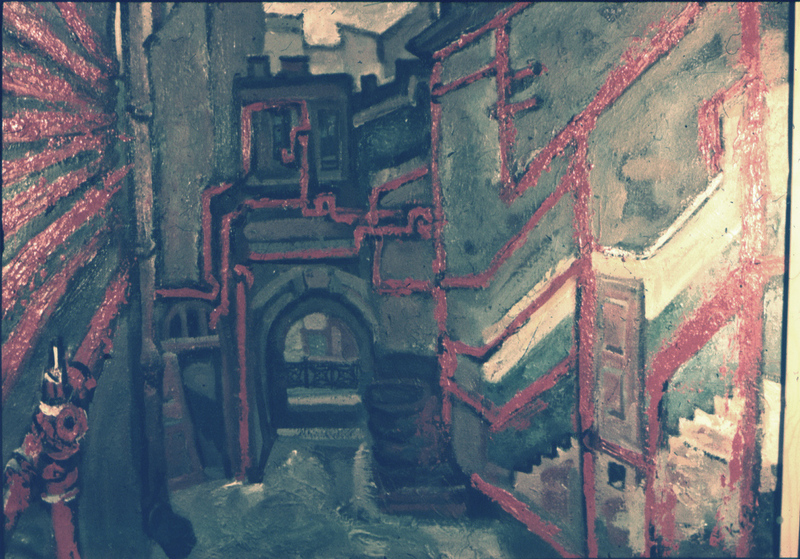This artwork depicts a stylized and abstract interior of an industrial building or alleyway. The scene is dominated by an archway at the far end, under which a gate is visible. The building's structure features numerous geometric shapes and angular lines, with several circular lines suggesting pipes running along the walls. These pipes, represented by vibrant red lines, stand out against the predominantly black, gray, and green surfaces.

The left side of the image has a distinctive green wall and an exposed pipe, reinforcing the industrial aesthetic. Shades of black, gray, tan, and white add complexity to the walls, while horizontal red lines create a cohesive visual thread. The ground appears to be either concrete or possibly water, adding to the ambiguity and abstract nature of the piece.

Details such as a graffiti-like depiction of stairs on the right wall and scattered horizontal red lines resembling pipes enhance the vibrancy and depth of the environment. The combination of these elements, including the green floors and the archway leading to the gated entrance, crafts a dynamic and intriguing representation of an industrial plant or urban alleyway.